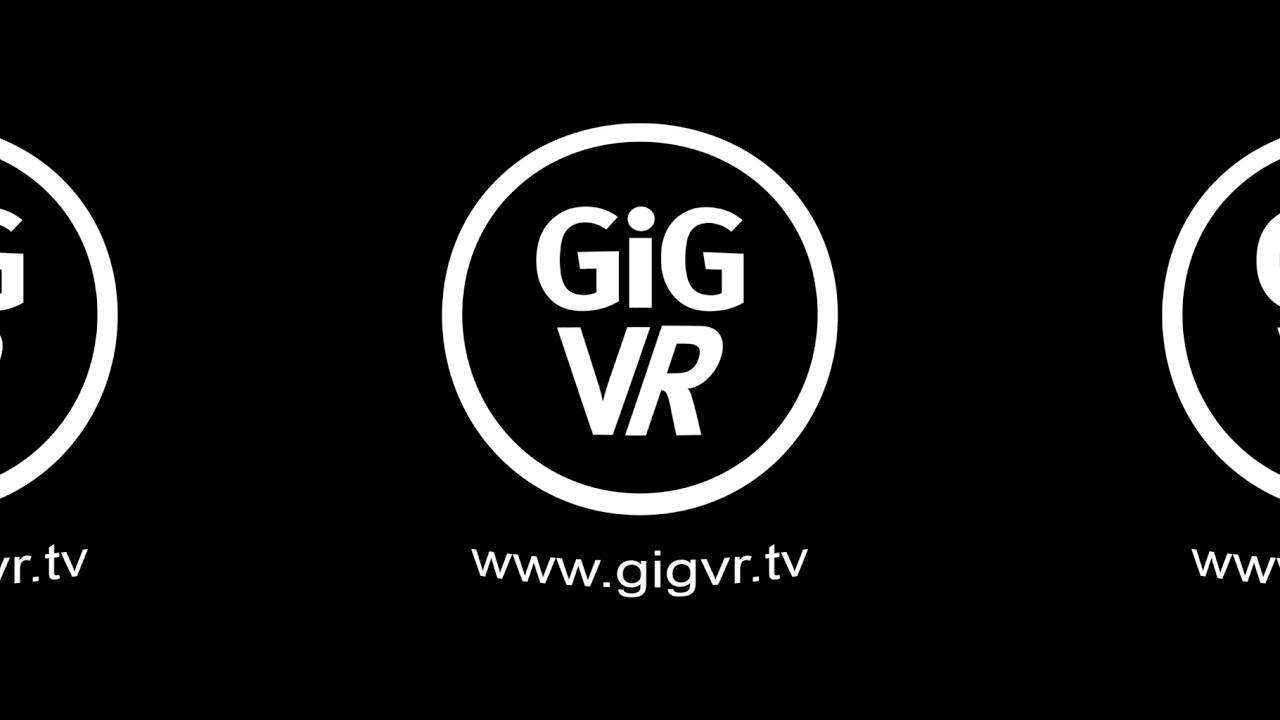The image features a bold, repeating logo set against a solid black background. Dominating the center is a large white circle, inside of which are the letters "GIG" on the top line, formatted as capital G, lowercase i, capital G, and directly beneath it, "VR" in capital letters. Beneath this text, within the circle, is the web address "www.gigvr.tv" also in white font. This central logo is mirrored on both the left and right sides of the image, but the outer logos are cut off, showing only partial circles and a fragment of the web address, enhancing the bold, symmetrical aesthetic of the design. The overall effect suggests a dynamic, perhaps digitally-enhanced visual meant for use as a wallpaper or a video screenshot.